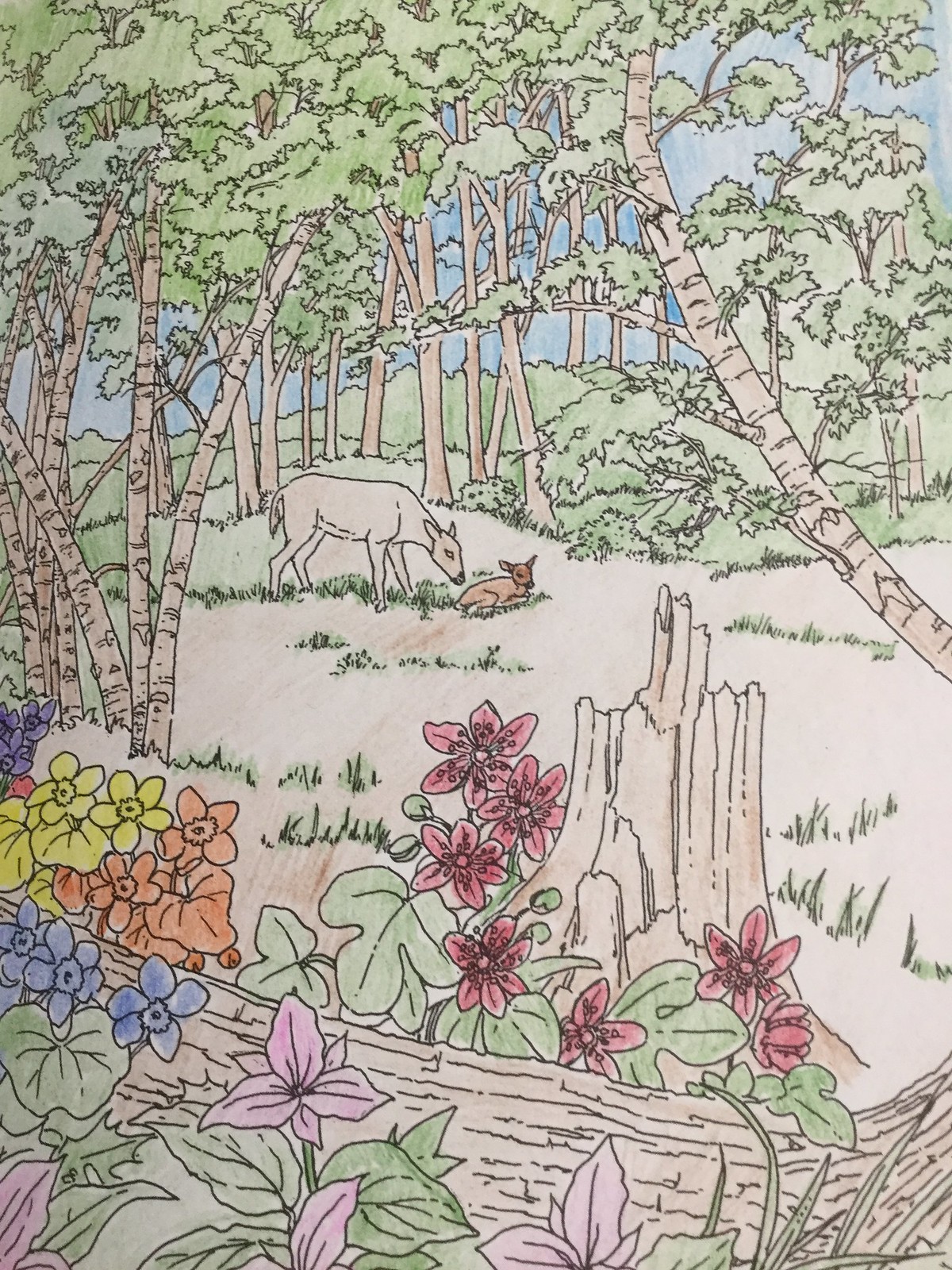The image depicts a serene forest clearing, vividly brought to life by someone’s coloring efforts. At the heart of the scene is a tender moment between a mother deer and her fawn. The fawn, colored in a delicate light brown, rests peacefully in the sporadically shaded grass. Its mother, though largely uncolored, stands protectively over it, gently sniffing her young. 

In the foreground, a fallen tree trunk, yet to be colored, lies adjacent to a brown tree stump. Surrounding this fallen trunk are clusters of brightly hued flowers in shades of yellow, orange, purple, and blue, accompanied by green foliage. 

The setting is further enriched by the presence of additional trees with rugged brown trunks and lush green canopies, extending into the background where low hills rise gently. Above, the sky stretches out, colored a soft, calming light blue, completing the picturesque natural tableau.